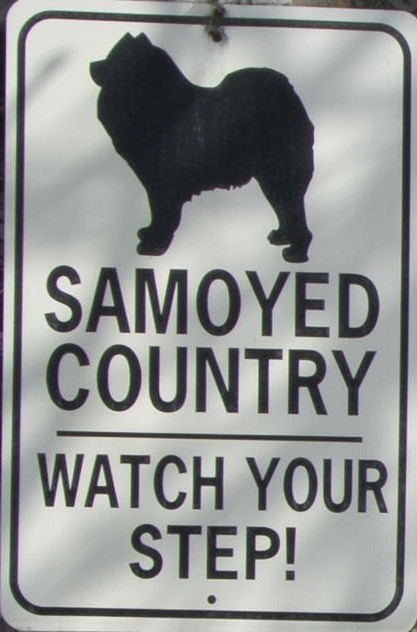This vertical rectangular metal sign features a distinctive design with a white background and a black border set within a thin white outer edge. At the top of the sign, there is a bold, monochromatic silhouette of a Samoyed dog facing left. Directly below the silhouette, large, bold black letters proclaim "Samoyed Country." A horizontal line separates this text from another message below it, which is printed in a slightly smaller all-caps font: "WATCH YOUR STEP." The sign exudes a classic, no-nonsense aesthetic with its white base, black silhouette, and striking black typography, emphasizing clarity and readability.